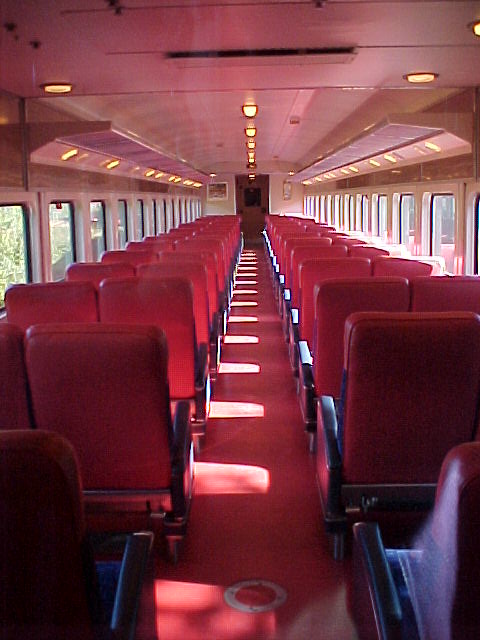This image captures the interior of a train car with detailed emphasis on its design and components. Each row in the train car consists of four red seats, divided by a central aisle, with two seats on either side. Adjacent to every seat, there is a window that allows natural light to filter in. The train car extends back through many rows of these red seats, and the floor is covered in matching red carpeting. A row of lights runs along the middle of the ceiling, complemented by additional lights along the interior sides, suitable for reading or illumination. At the far end of the train car is a brown door with a small, dark-tinted window that provides a glimpse of the outside, potentially showing trees or grass. Flanking this door are pictures on each side. The overall ambience of the train car is well-lit and orderly, with consistent red and brown hues contributing to its cohesive design.